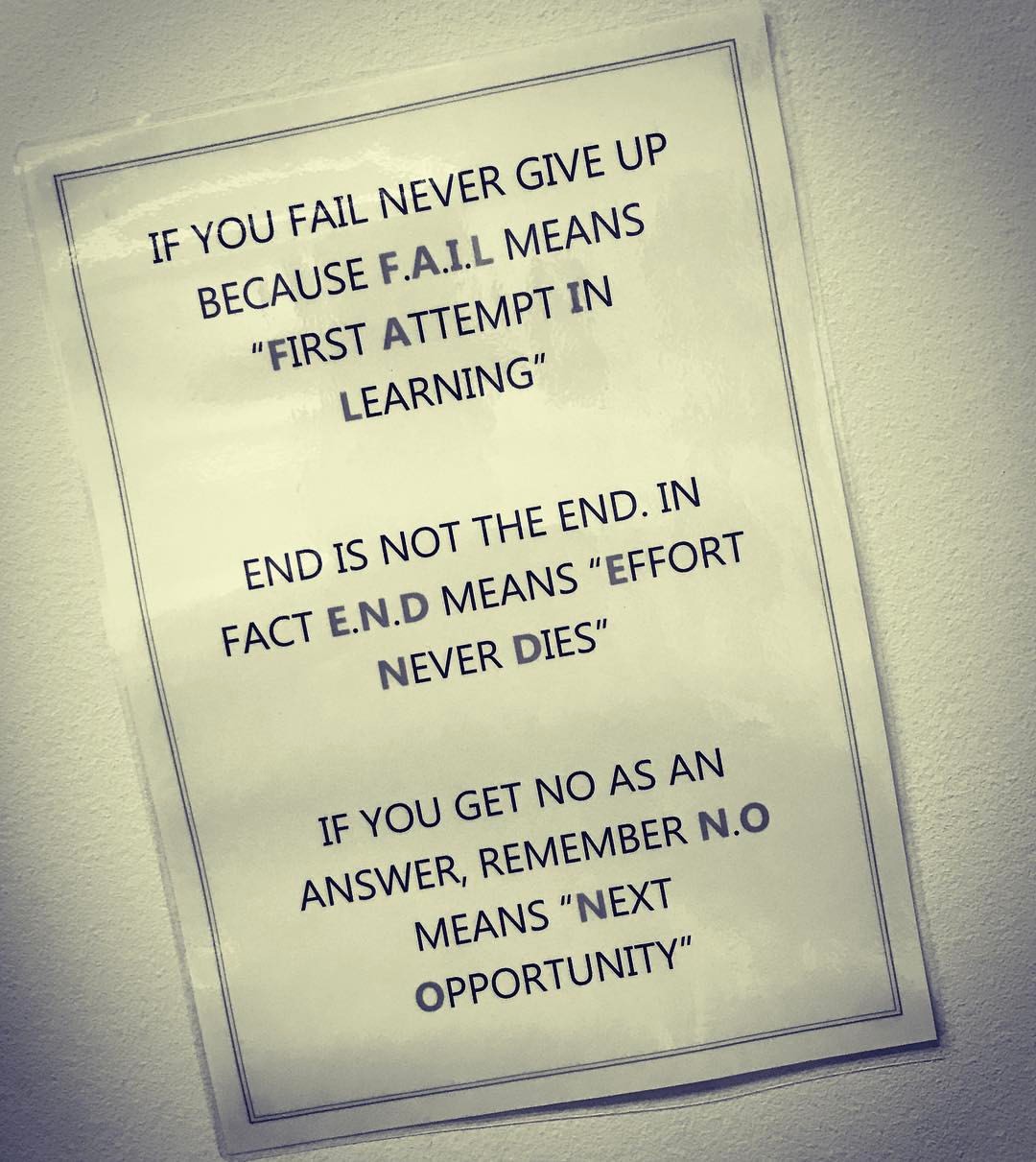The image features a laminated white poster with black and gray text displaying a motivational message. Situated indoors against a stone wall, the poster is slightly off-center and positioned at a diagonal angle, giving it a crooked appearance. The motivational text reads in all capital letters: "If you fail, never give up, because FAIL means first attempt in learning. End is not the end. In fact, END means effort never dies. If you get NO as an answer, remember NO means next opportunity." The setting suggests a place of work, aiming to inspire perseverance and optimism.